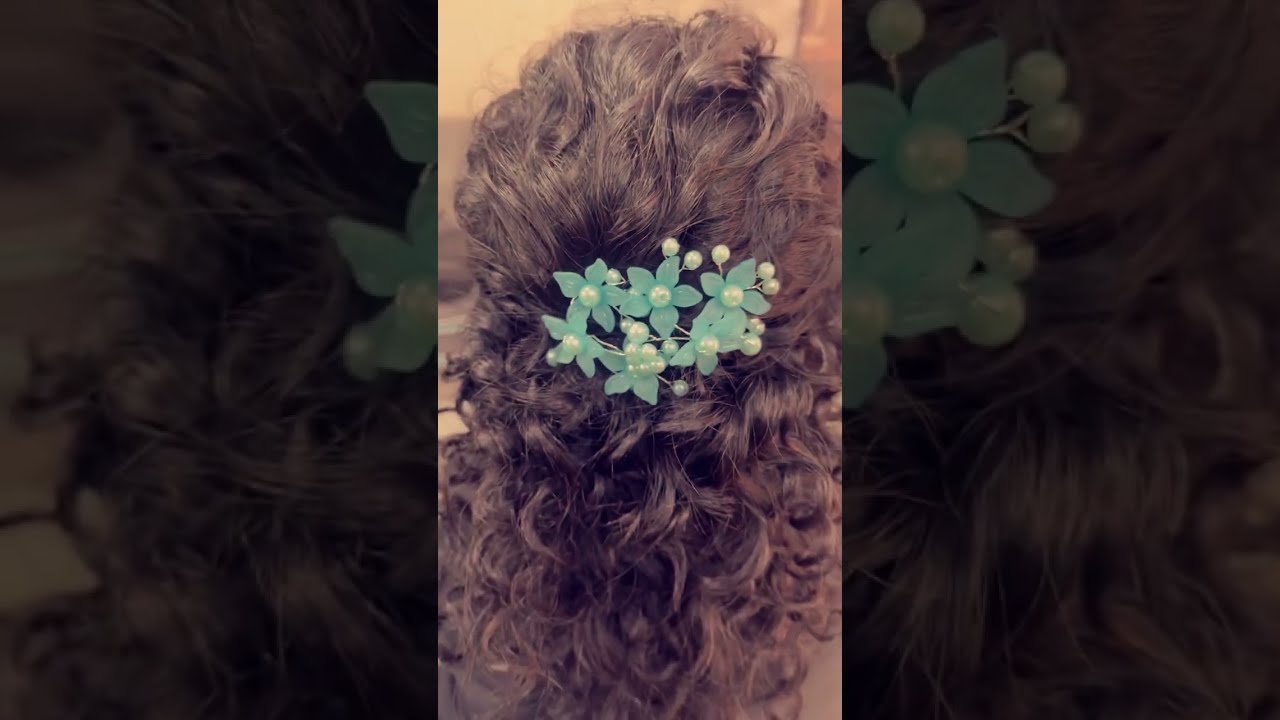The image is a detailed photograph split into three parts, focusing on the back of a woman’s head with luxuriant, dark brown, wavy, and curly hair cascading down. Dominating the center frame, her hair is adorned with a decorative pin featuring six teal flowers with white pearls at their centers and additional pearls scattered among the flowers. A light tan wall serves as the background, with a small portion visible near the top. The two outer rectangles are zoomed-in sections of her hair, reflecting parts of the central image. The left side shows an enlarged view of the curly hair with a glimpse of the green flowers, while the right side highlights the wavy hair with a flower adorned with white beads in the upper left corner.